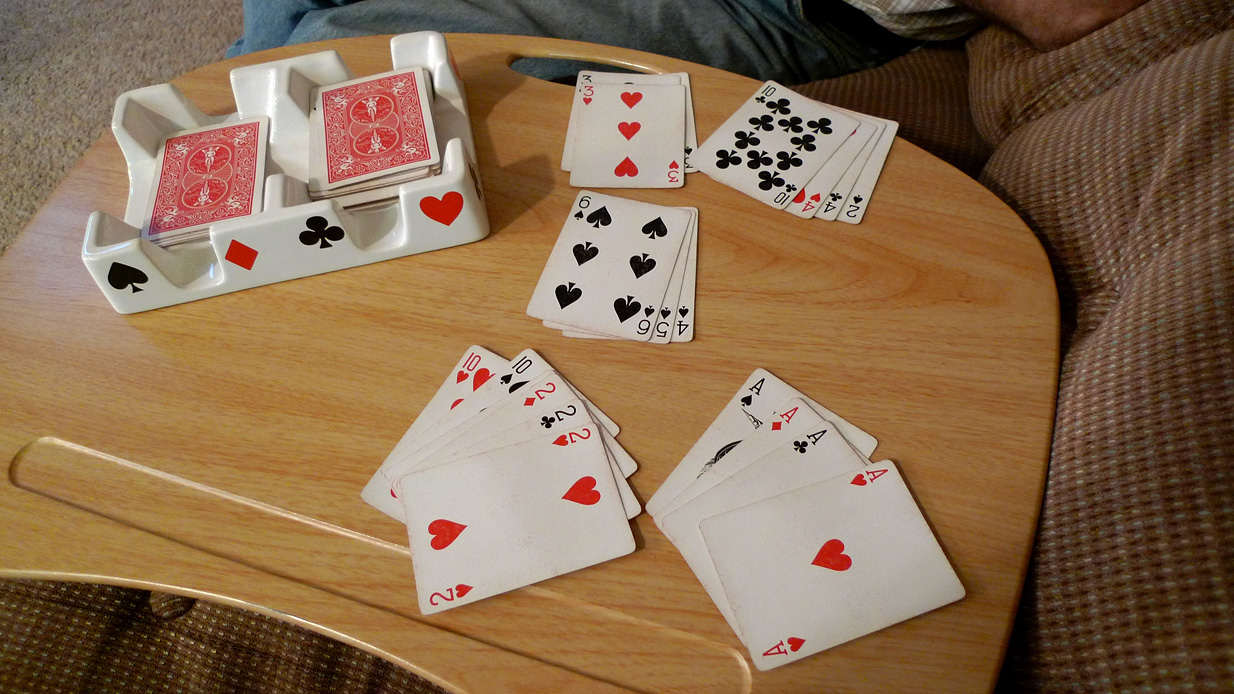The photograph captures a cozy living room scene. In the upper left corner, the plush brown carpet is visible. Dominating the right side of the image is a couch upholstered in brown fabric. Centrally positioned in the scene is a natural wood tray table, rectangular in shape with curved top and bottom edges, featuring an open handle area at the top. 

On the tray table, in the upper left, sits a white rectangular container divided into two sections, adorned with black spade, red diamond, black club, and red heart symbols. Inside the container are two decks of cards, each with red tops and their cards facing down. 

Spread out next to the container are five neat stacks of playing cards. The upper left stack reveals a three of hearts, beside which is a ten of clubs. Directly beneath the three of hearts stack, there is a six of spades. Another fan of cards shows the hand of the player, starting with a two of hearts, followed by a ten of hearts, a ten of spades, a two of diamonds, a two of clubs, and concluding with another two of hearts. Adjacent to this hand is a separate set of four aces displayed: the ace of spades, ace of diamonds, ace of clubs, and ace of hearts.